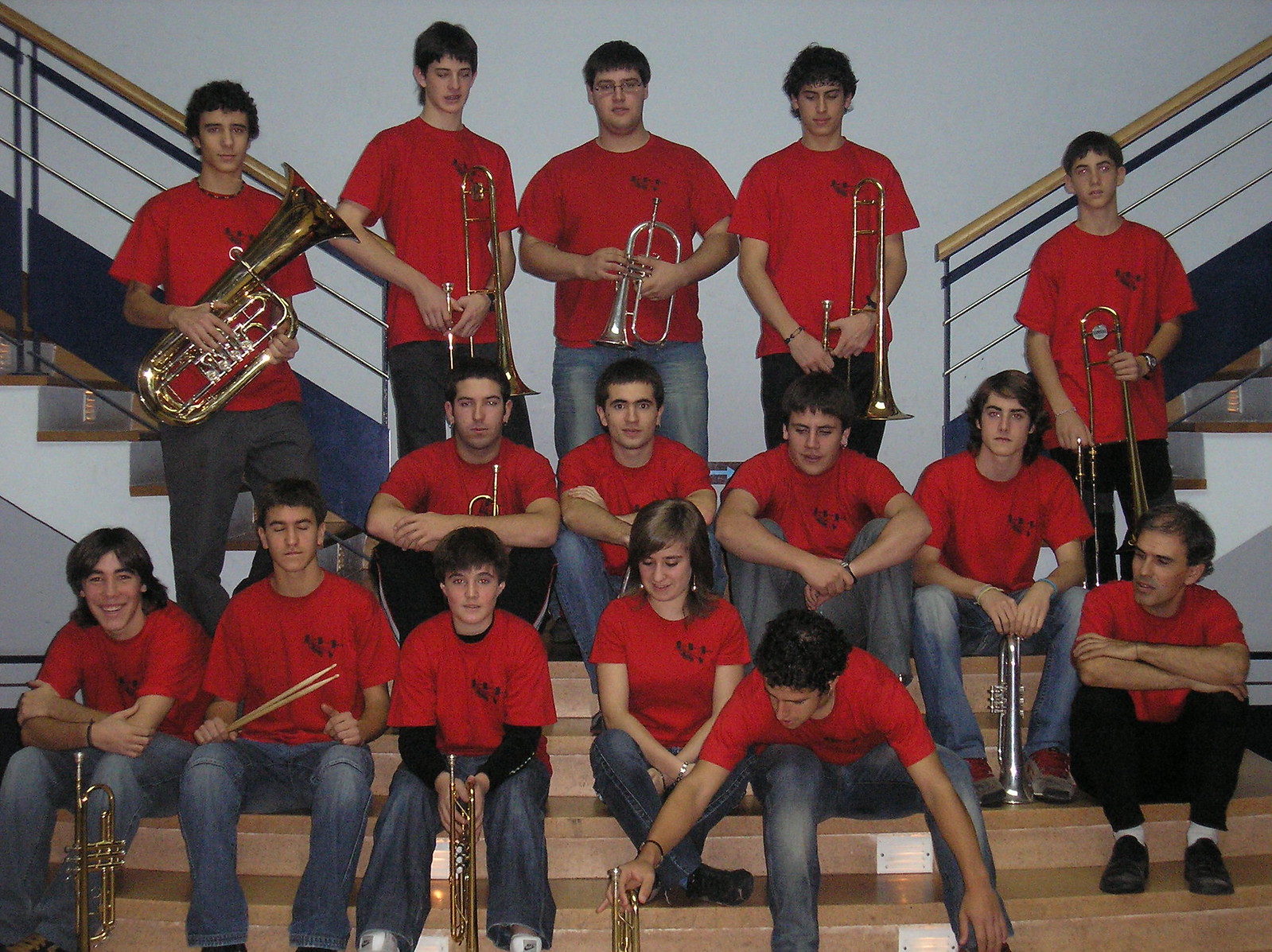This indoor photograph captures a group of young people, likely middle or high school students, who appear to be members of a band. They are arranged in three rows on wooden risers with white sides, flanked by staircases leading up to the right and left. The backdrop is white, providing a stark contrast to their red shirts adorned with a logo, and various shades of denim jeans. In the top row, a gentleman prominently holds a gold tuba, flanked by individuals with saxophones and other brass instruments. The middle row features more students with additional saxophones, while the bottom row includes a mix of instruments, notably a silver clarinet and various trumpets or cornets. One of the bottom row individuals is holding a pair of drumsticks. All members, except for a few, are holding their instruments, and a person in the middle is notably bending over with a hand on a saxophone. The entire scene showcases these young musicians in a structured display, embodying their collective identity through uniform attire and instrumental presence.